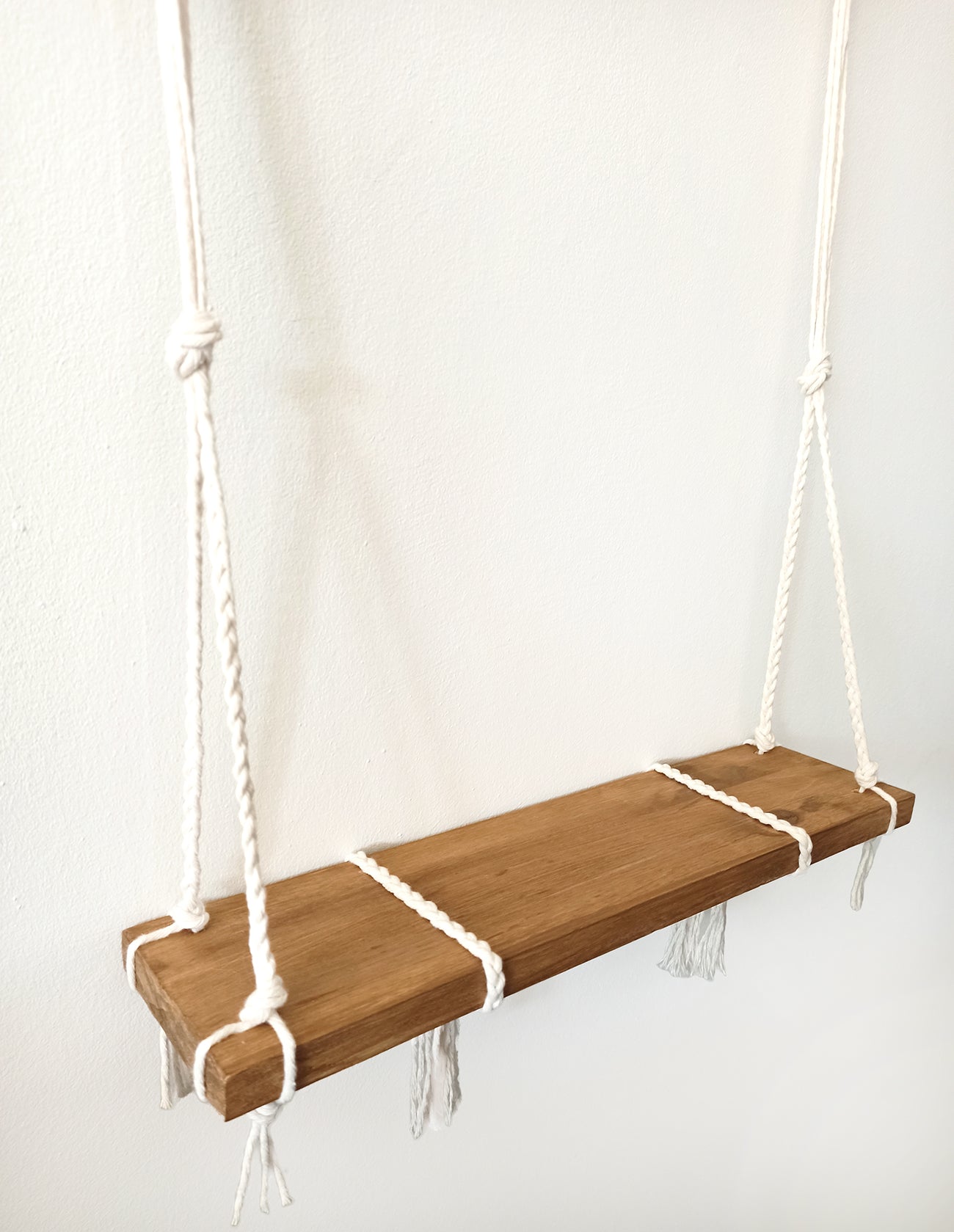The image features a simple yet charming wooden swing set against a white wall. The swing consists of a light brown wooden board suspended by sturdy, white braided ropes. These ropes are securely tied with knots at each of the four corners of the board, with additional white cords running vertically over the center for balance and stability. The tails of these ropes hang down beneath the board, adding to the aesthetic detail. The background is very pale, almost white, which creates a slight shadow of the swing and ropes against the wall, enhancing the serene and minimalistic composition of the scene.